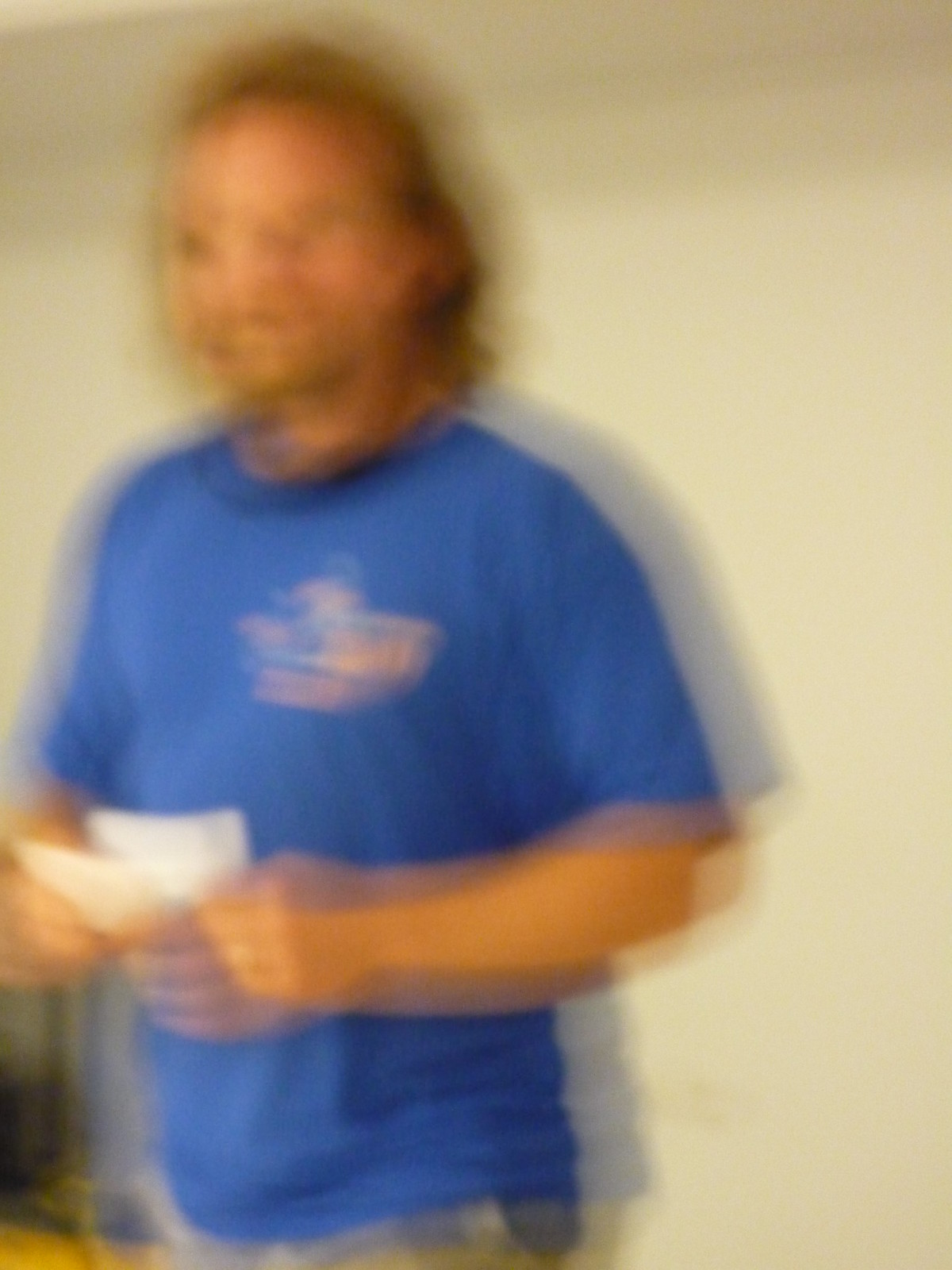In the extremely blurry image, a man of light complexion with a mustache and goatee is depicted. His hair, which appears to be either blonde or red, is styled into a mullet—it is longer at the back and slightly shorter on the sides. He is seen wearing blue jeans and a blue shirt that bears an indistinguishable graphic. The subject is holding a white card, presumably reading aloud from it. The backdrop consists solely of a plain white wall. Due to the extensive motion blur affecting both the subject and the person who took the photo, finer details of the man's facial features and the graphic on his shirt remain unclear.